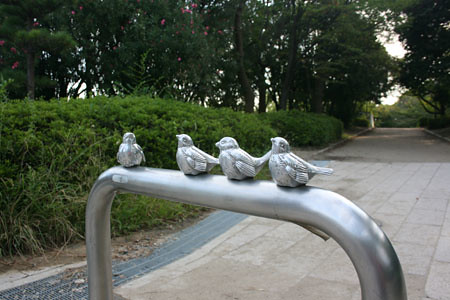The image captures a detailed scene at the end of a long, beautifully paved driveway or walkway, adorned with beige stone tiles and lined with gray brick. Dominating the foreground is a shiny chrome metal railing, resembling the end of a bicycle rack, bent into a semi-circular arch. Atop this arch sit four small metal bird sculptures, all facing the same direction. The birds vary in size, with three situated close together and the fourth slightly apart on one edge. They are chubby and arranged in a progressive size order from right to left. The scene is set outdoors on an overcast day, surrounded by lush greenery. Tall trees with thick green leaves and large green shrubs line the path, creating a serene, park-like atmosphere. Additionally, a discreet green storm grate runs along the left side of the walkway, designed for rainwater drainage. The entire setting suggests a tranquil, maintained area, possibly the entrance to a private home or a mansion.